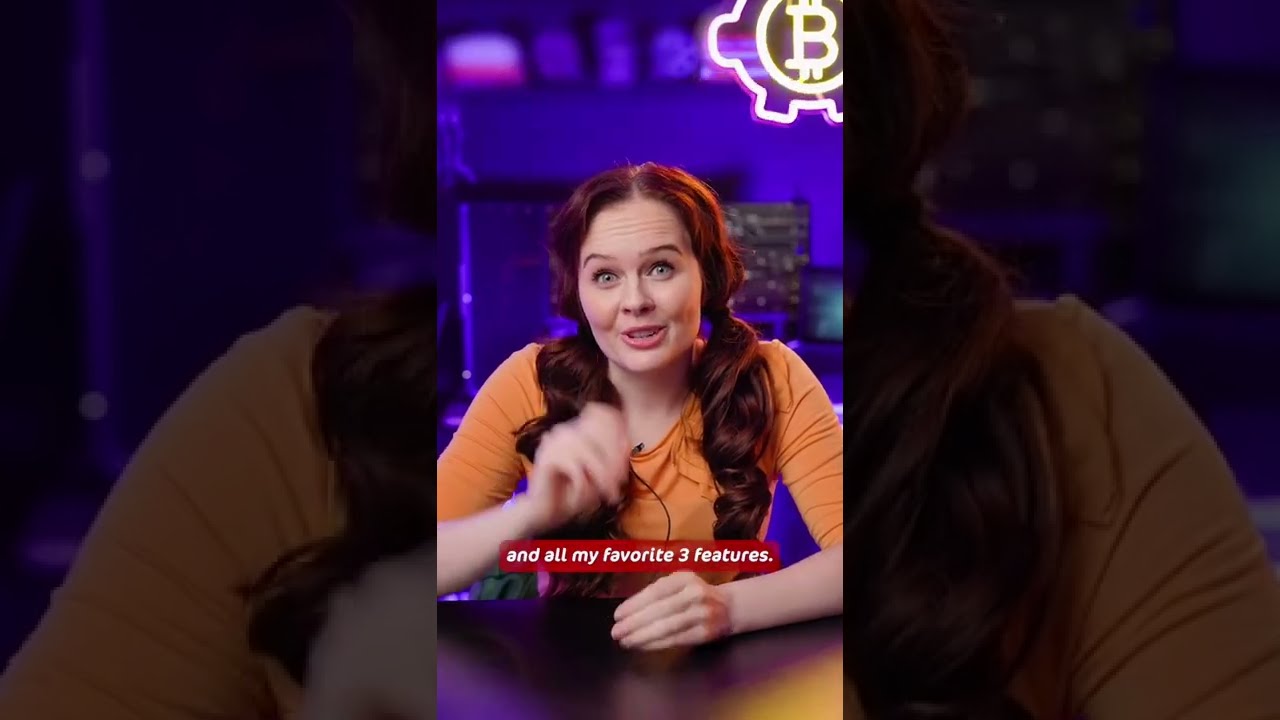In this image, we observe a well-lit scene appearing to be a still shot from a TikTok video or a similar content creation setting. Central to the image is a smiling woman with fair skin, blue eyes, and vibrant red hair styled in curly pigtails. She is dressed in an orange long-sleeve shirt, pushed up to her elbows, and has a little microphone clipped to her collar, with a black cord hanging down. The woman is positioned chest up, with her left hand resting on a dark wooden table at the bottom of the image.

In the background, the setting features a blue and pink illuminated room, partially obscured and blurry, giving a sense of depth. On the top right corner of the image, a prominent yellow neon sign displays the Bitcoin logo—a capital "B" with dollar signs enclosed in a circular cog design. Over the woman’s left shoulder on the right side of the image, there appears to be a screen which blends into the rest of the background.

At the bottom of the image, a red bar displays white italicized text reading "and all my favorite three features". This combination of elements, from the detailed backdrop to the specific features of the subject, suggests a meticulously arranged composition aimed at creating engaging visual content.